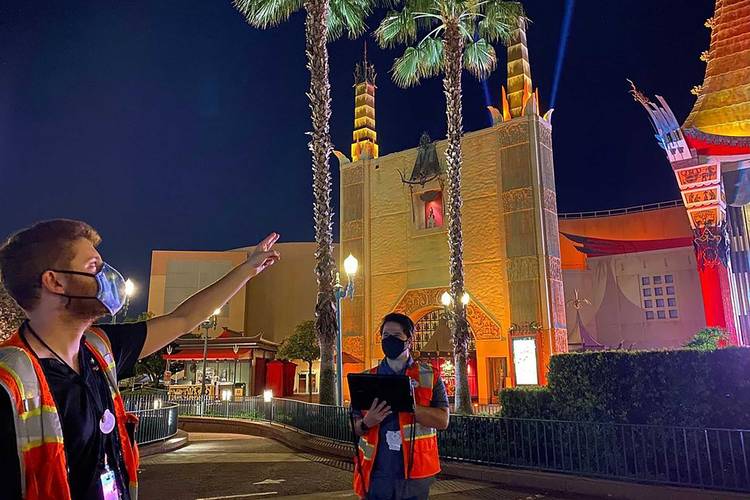In this horizontally aligned rectangular picture taken at an amusement park, the scene captures a setting just turned evening with a very dark blue sky. Central to the background are two tall palm trees with brown stems and a mix of green and brown leaves at the top. The focal point is the entrance to the theme park, highlighted by a large, illuminated, light yellow building that appears to take up an entire block. This building features a large, three-story, golden brown arched doorway flanked by beams and turrets, along with a partially visible triangular-shaped roof on the right side. The roof is supported by red beams.

In front of the building, two workers are visible. On the left side, one worker with short brown hair and facial hair is wearing a red or orange and yellow safety vest over a dark shirt. He has a lanyard with a name tag around his neck, a mask on his face, and is pointing towards the building with his left hand. In the center, another man with black hair, wearing a black mask and similar safety vest, is holding what appears to be an iPad in his right hand. Both workers are near a metal railing that section off the pathway, which is lined with neatly trimmed hedges and bordered by a long black fence with vertical bars. Additional shrubs are visible behind the right side of the fence, enhancing the landscaped area.